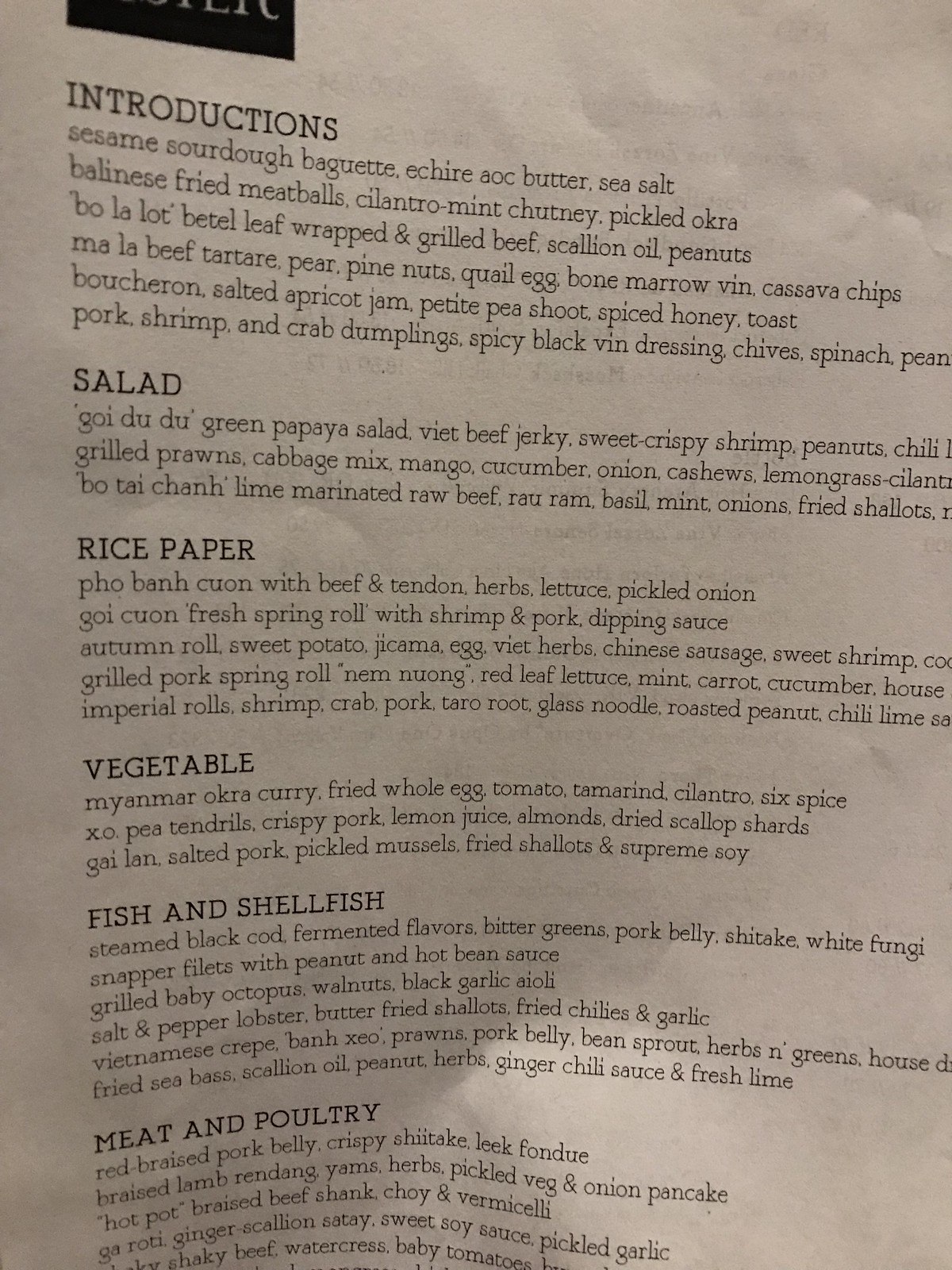**Intriguing Ingredients Sheet**

A crumpled and slightly creased white piece of paper, seemingly handled quite a bit, showcases an array of delectable ingredients. At the top left, there is a partial view of a black rectangular shape with white writing, the details of which remain obscured. Below this mystery rectangle, the word "INTRODUCTIONS" boldly stands out in all caps. This section lists:

- Sesame Sourdough Baguette
- Ikir AOC Butter
- Sea Salt
- Balinese Fried Meatballs
- Cilantro Mint Chutney
- Pickled Okra
- Bola Lact
- Betel Leaf Wrapped Grilled Beef
- Scallion Oil
- Peanuts
- Mala Beef Tartare
- Pear
- Pine Nut
- Quail Egg
- Bone Marrow
- Vean Cassava Chips
- Boucheron
- Salted Apricot Jam
- Petit Pea Shoot
- Spiced Honey Toast
- Pork, Shrimp, and Crab Dumplings
- Spicy Black Bean Dressing
- Chives, Spinach, Peanuts

The next section, titled "SALAD" in all caps, details some visible ingredients before the text becomes illegible:

- GOI DU DU (Green Papaya Salad)
- Viet Beef Jerky
- Sweet Crispy Shrimp
- Peanuts
- Chili
- Grilled Prawns
- Cabbage Mix
- Mango
- Cucumber
- Onion
- Cashews
- Lemongrass
- Cilantro
- Lime Marinated Raw Beef
- Rau Ram (Viet Coriander)
- Basil
- Mint
- Onions
- Fried Shallots

Following "SALAD," the headers continue with "RICE PAPER," "VEGETABLE," "FISH AND SHELLFISH," and finally "MEAT AND POULTRY" in all caps at the bottom. Under "RICE PAPER," the sheet reads:

- Pho Van Quang with Beef and Tendon, Herbs, Lettuce, Pickled Onion
- Goi Quang, Fresh Spring Roll with Shrimp and Pork, Dipping Sauce
- Autumn Roll, Sweet Potato, Jicama, Egg, Viet Herbs, Chinese Sausage, Sweet Shrimp
- Grilled Pork Spring Roll, Nem Nuong, Red Leaf Lettuce, Mint, Carrot, Cucumber
- House Imperial Rolls, Shrimp, Crab, Pork, Taro Root, Glass Noodle, Roasted Peanut, Chili Lime

While the text becomes incomplete at several points, the essence of a meticulously curated menu rich in diverse flavors and culinary traditions is vividly present.